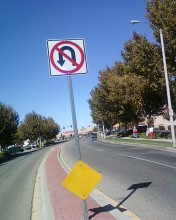The photograph captures a street sign positioned on a silver metal post situated in the middle of a brick-paved median. The median separates two roads that run parallel on either side. At the base of the post, there's an empty yellow diamond-shaped sign. Above it, there is a standard "No U-turn" sign, which is a white square with a black U-turn symbol overlaid by a red circle with a diagonal line through it, indicating that U-turns are prohibited. The background consists of lush green trees and a clear, blue sky with no clouds, providing a stark contrast to the structured elements in the foreground.